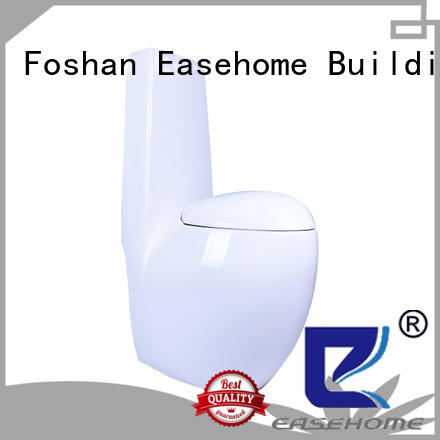This image is an advertisement flyer featuring a sleek, futuristic-looking, white toilet that closely resembles an upside-down Apple AirPod in shape. The toilet is centrally placed on a plain white background, with no additional details behind it. A distinctive gray border with a swoosh pattern at the bottom and a corner cut-off at the top left frames the entire image. Above the toilet, the incomplete text "Foshan Ease Home Buildee" is prominently displayed, partially cut off by the border. Below, a red seal reads "Best Quality," and to its right, a blue logo with the name "Ease Home" further identifies the brand.